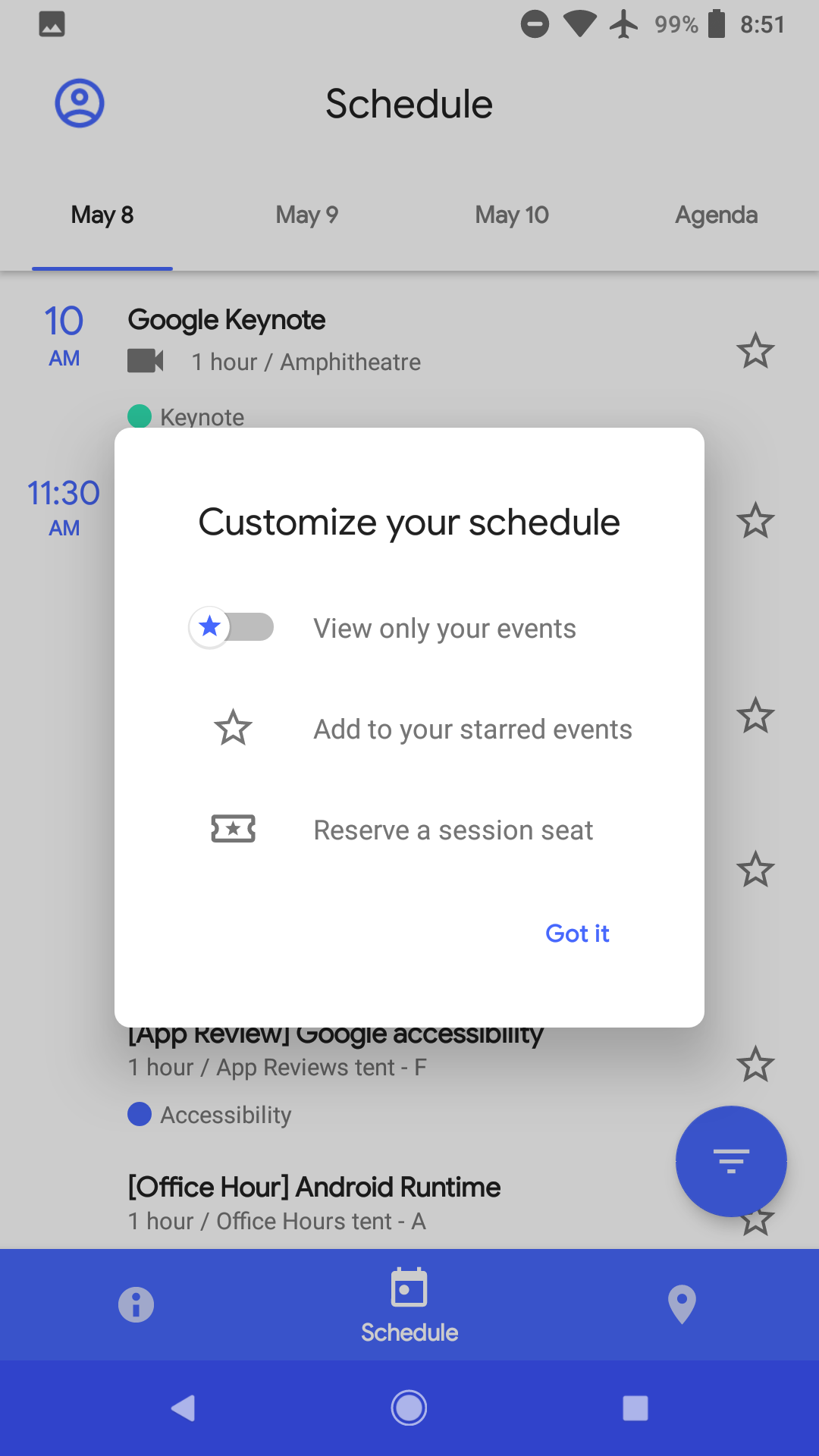A detailed screenshot of a smartphone's calendar app displaying a series of scheduled events for May 8th. The agenda begins at 10 a.m. with an entry for a "Google Keynote." Below this, the schedule entries from 11:30 a.m. are partially obscured by a pop-up window, which appears to be a tutorial or introductory guide for customizing the calendar settings. The title of the pop-up reads "Customize Your Schedule," and it lists three options in bullet points: "View only your events," "Add to your starred events" accompanied by a star icon, and "Reserve a session seat" illustrated with a ticket icon. At the bottom of the pop-up is a blue clickable button labeled "Got it," intended to close the tutorial and return the user to their full schedule. The presence of the pop-up suggests that this might be the user's first time accessing the calendar or that the app has recently been updated. The rest of the calendar page is blurred or hidden, emphasizing the new feature tutorial initiated by the app.